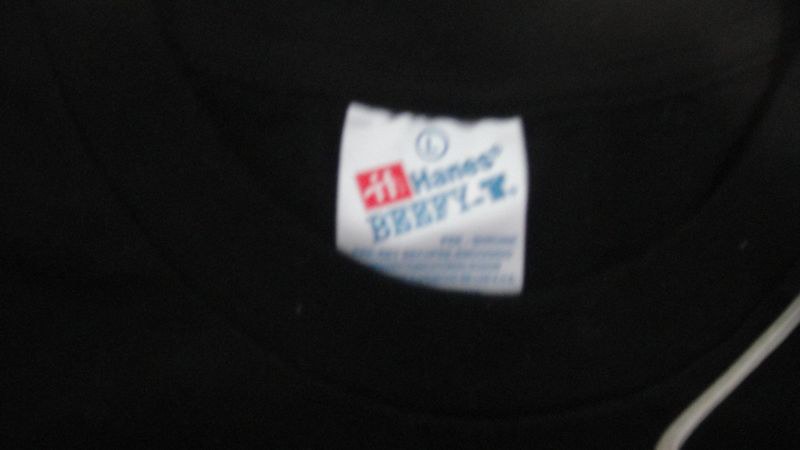This image is a close-up, albeit very blurry, of the tag on a black Hanes Beefy T-shirt. Dominating the frame, the white square tag is positioned on the inside collar at the back of the shirt. The tag prominently features a teal circle with an "L" at the top, signifying the size large. Below this, there is the angled Hanes logo: a red rectangle with a white "H" and the word "Hanes" in teal beside it. Further down, also angled, are the words "Beefy T" in teal, followed by some indistinct lettering at the bottom. The right side of the tag is curled under, while the bottom left edge appears folded back. Additionally, a white stripe or cord runs diagonally across the bottom right corner of the image, contrasting against the black background of the t-shirt.